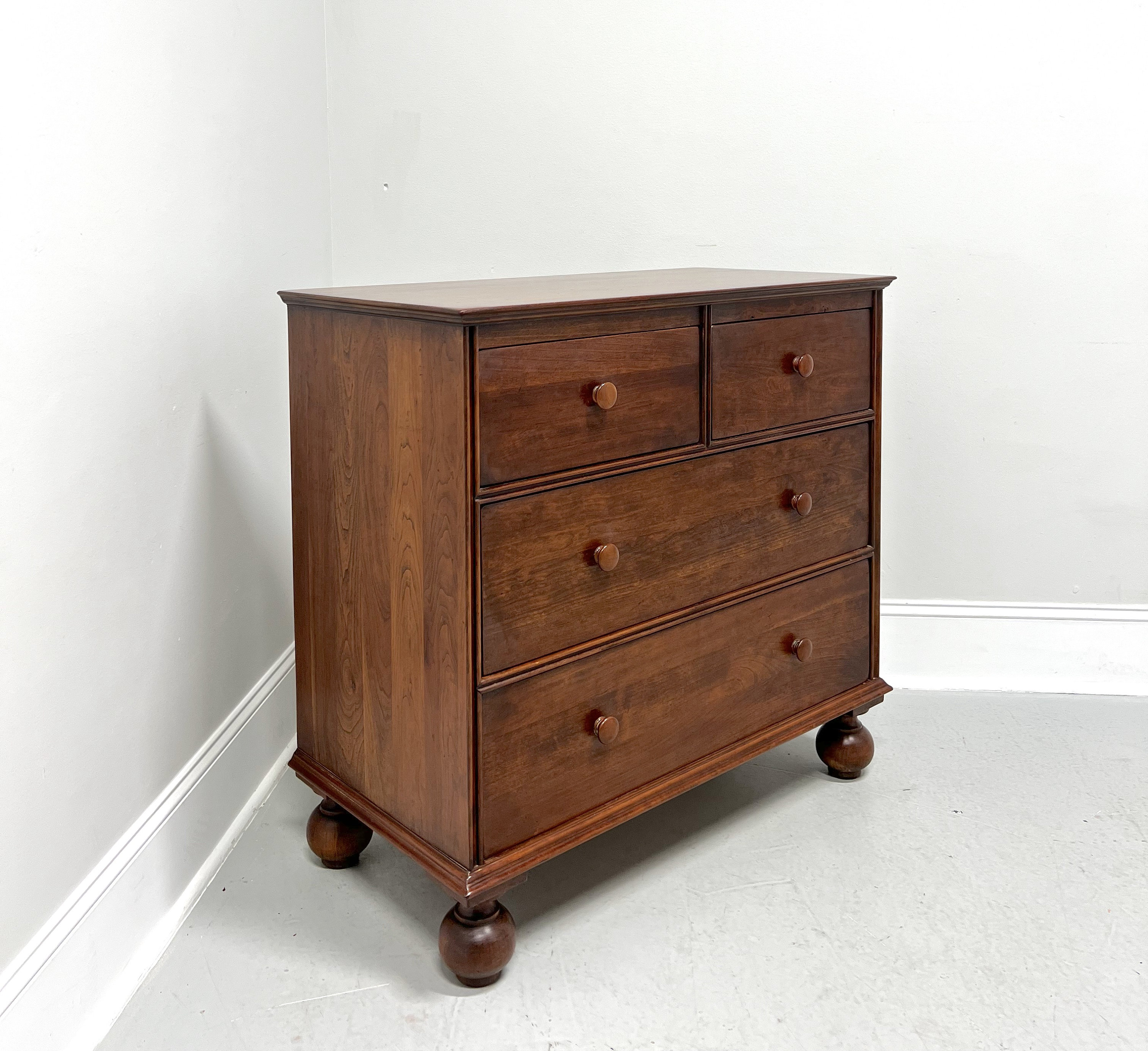In the corner of an empty room with light gray walls and a gray linoleum floor, stands an antique, medium-sized dresser made of dark brown wood that resembles walnut. The room features a thick, colonial style white baseboard with quarter round trim. The dresser itself has a simple yet elegant design, comprising four drawers: two large, full-width drawers at the bottom and two smaller, half-width drawers at the top. It rests on four rounded, ball-like feet which elevate and protect it from the floor. Each drawer is adorned with single wooden button knobs, maintaining the dresser's antique aesthetic. The combination of the dark walnut finish and the minimalist design elements creates a charming piece that stands out against the sparse, neutral-colored room.